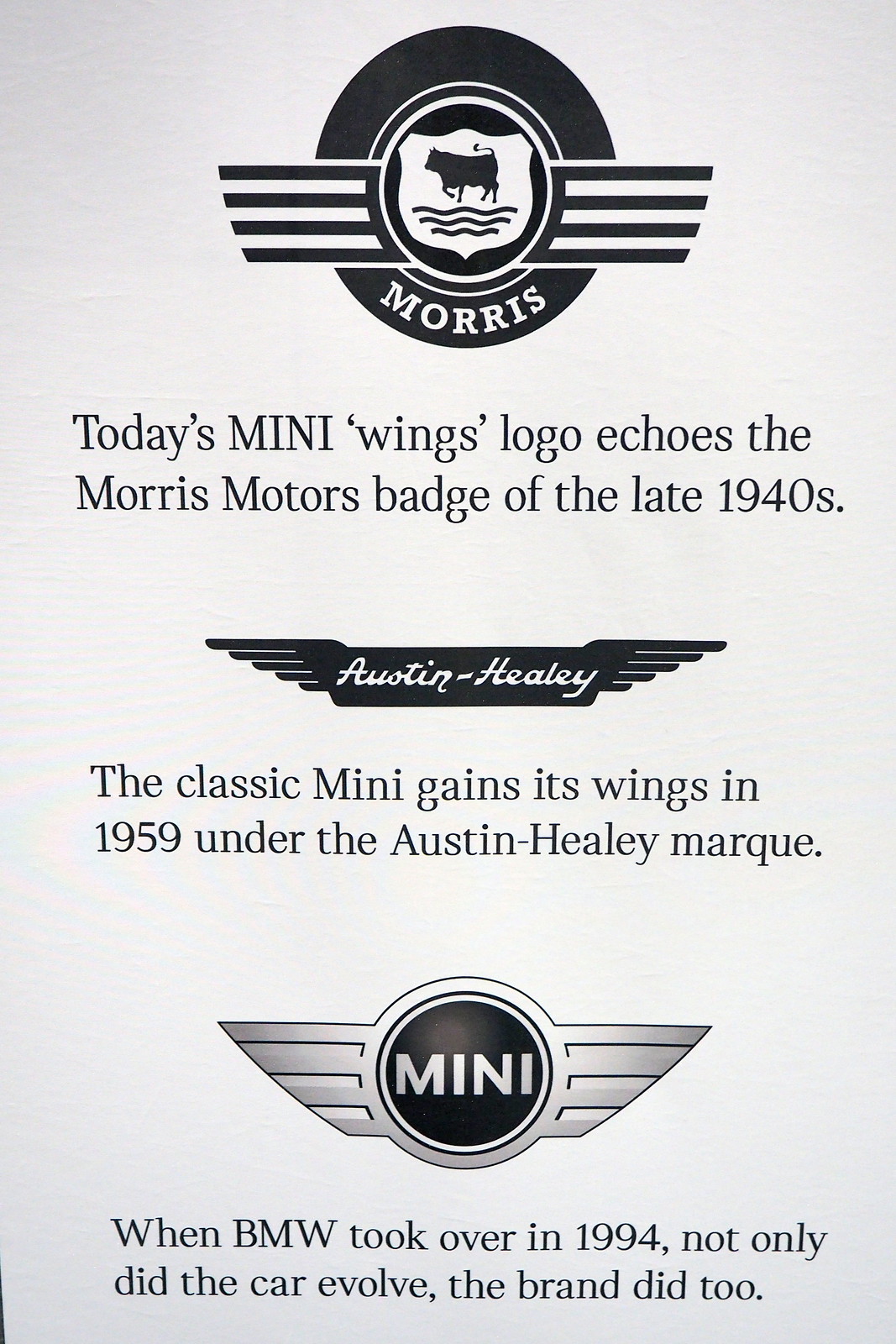The image is a vintage, black-and-white advertisement for the Austin Healey brand, featuring a transition of logos through time and emphasizing their connection to Morris Motors and Mini under BMW's ownership. At the top, there is a circular logo with a depiction of what appears to be a bull or cow, accompanied by lines beneath, and labeled "Morris," reminiscent of the Morris Motors badge from the late 1940s. Beneath this, the text notes how the modern "Mini Wings" logo takes inspiration from this historic badge. In the middle, the Austin Healey logo with its signature winged design is prominently displayed, marking the classic Mini's association with the Austin Healey marque since 1959. At the bottom, the updated Mini logo is shown, accompanied by text indicating that when BMW took over in 1994, both the car and the brand underwent significant evolution. The overall arrangement and monochromatic scheme give a clear and historical representation of the brand's legacy and transformation over the decades.